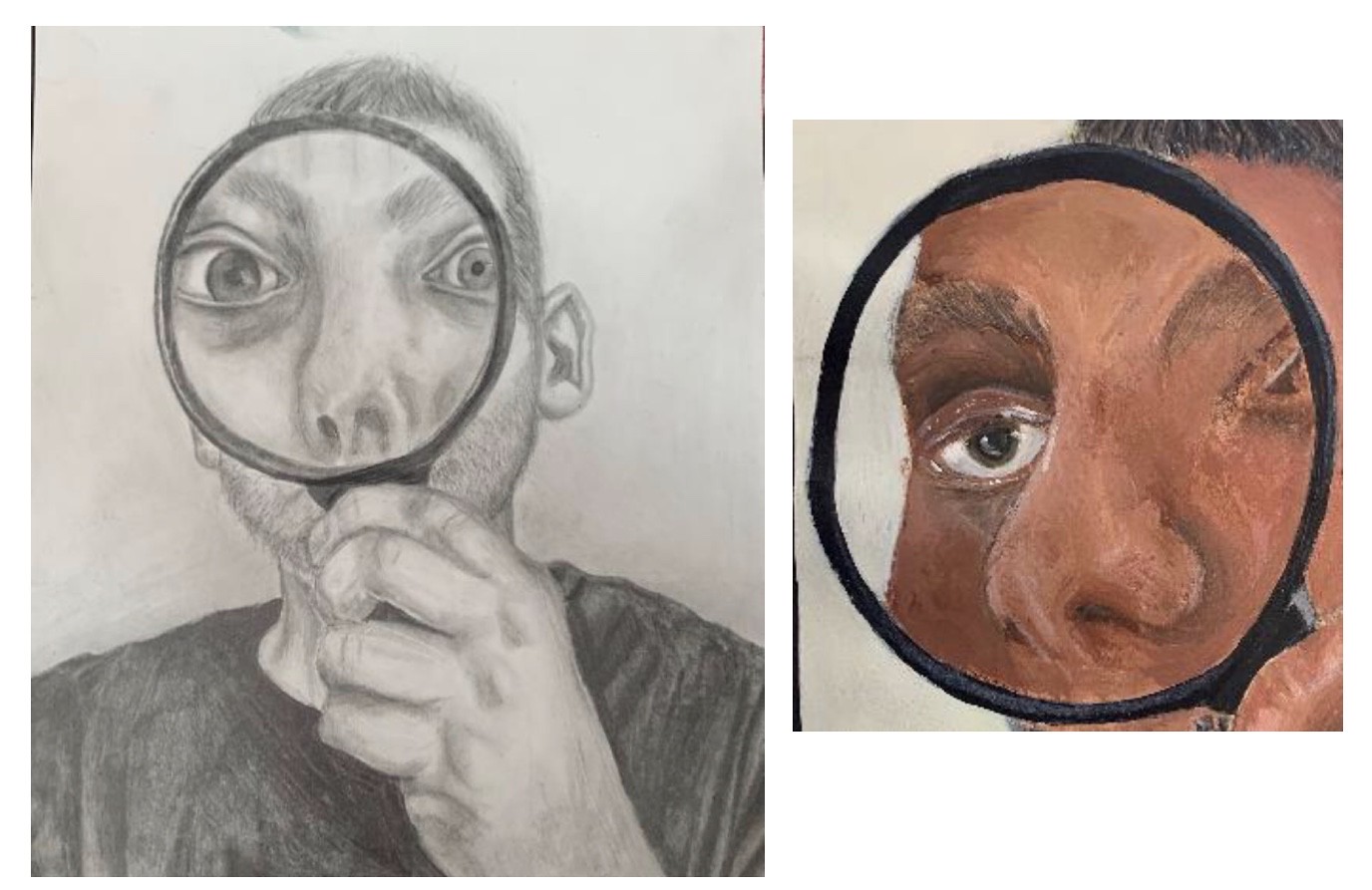The image consists of two side-by-side drawings. The drawing on the left is a full-sized portrait of a person, showing their face, part of their shoulders, and a small portion of their chest. The individual is depicted holding a magnifying glass in front of their face, through which their features are intricately magnified. The right-hand side drawing is a smaller, close-up depiction of the same scene, focusing solely on the face and magnifying glass. This zoomed-in version has more vibrant colors, with the skin tones being particularly well-defined.